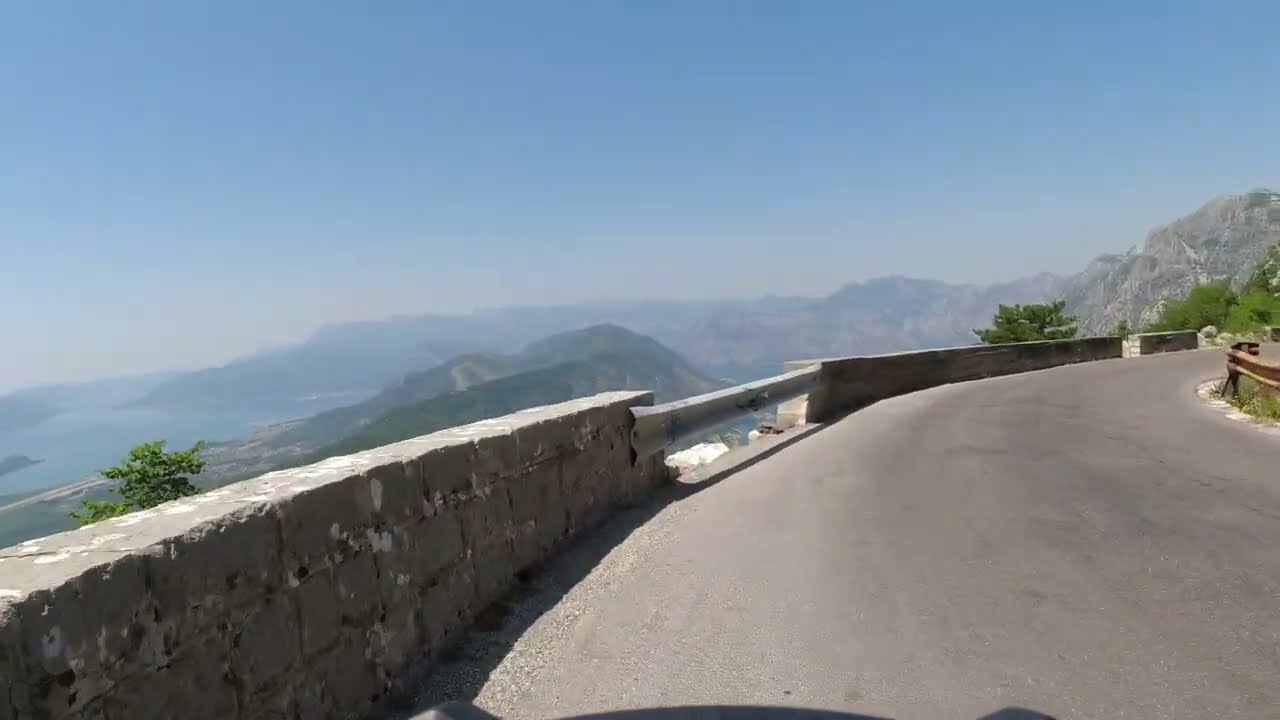The image captures a high-altitude mountain road, presumably in a historical European area, evident from the well-maintained stone and brick retaining walls and the car driving on the left side of the two-lane road. The road is pristine cement concrete with segments of brick walls that start from the bottom left and curve towards the center right, intersecting with metal guardrails at sections. The guardrails ensure continuous safety along the roadside, preventing any falling off the steep drop-offs. On the left side, there's a panoramic view of tan-colored, dry mountains showcasing some greenery and grey granite features, descending into a distant large body of water. The ambiguous water body, possibly a large lake or a coastal bay, is semi-shrouded in haze with a cloudy sky backdrop. Additionally, there's a hint of a town or buildings nestled by the coastline. The photograph seems to be taken from inside a vehicle, providing an expansive high-up perspective of the scenic landscape.